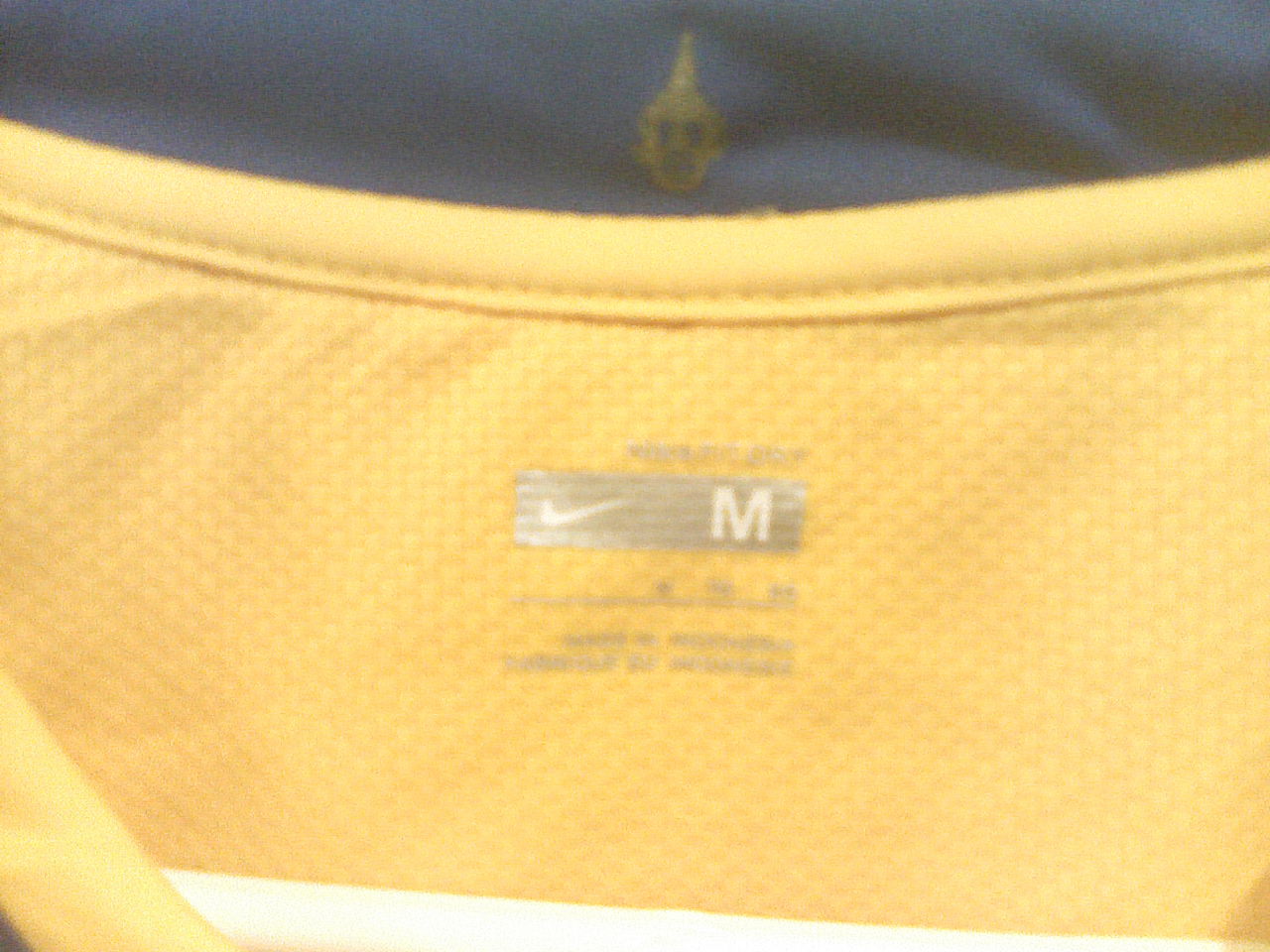The image displays the inside tag of a yellow shirt, crafted from a soft, cotton-like woven fabric. The tag prominently features the Nike logo, indicating the shirt is a size medium (M). Surrounding this yellow fabric, the shirt is placed on a blue background that showcases an illustration of a face adorned with a unicorn horn at the top. Additionally, a white element is visible at the bottom of the frame, adding contrast to the overall composition.